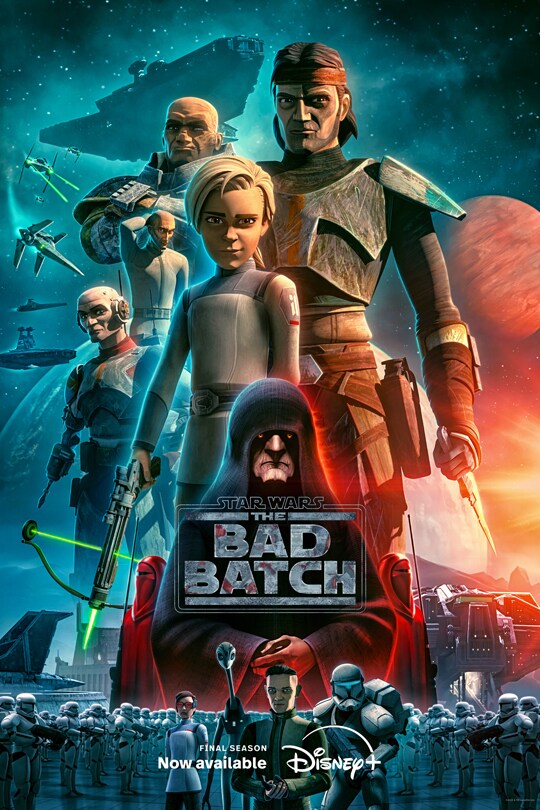This poster image is an advertisement for a TV show titled "The Bad Batch," now available on Disney+. The artwork features six distinct cartoon-like human characters, all of whom appear to be male. Among them, one stands out as a teenage figure. At the center of the image is an older man dressed in a hooded cloak, with only his nose, mouth, and chin visible. The bold text "The Bad Batch" is prominently displayed, indicating the show's title, followed by an announcement that it is currently streaming on Disney+.